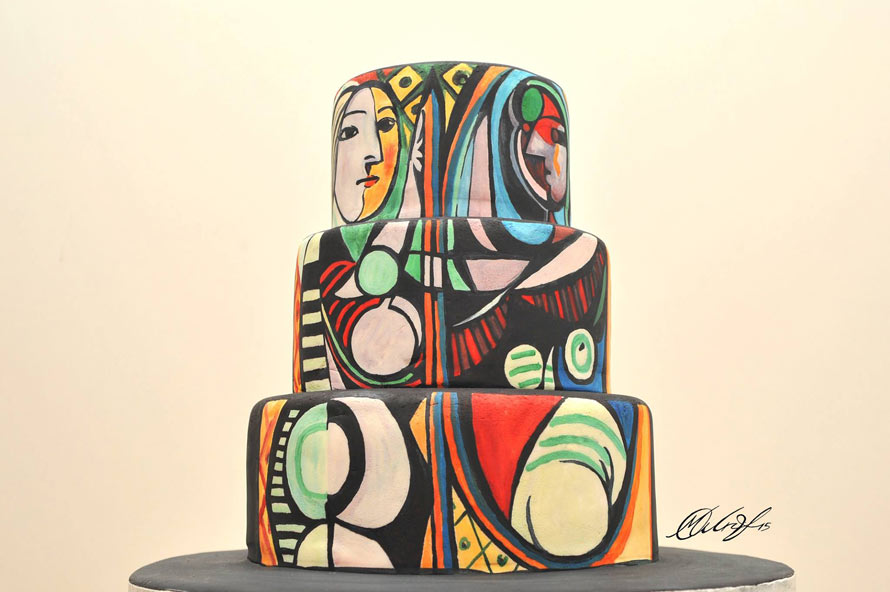The image is a detailed and abstract depiction of what appears to be a professionally crafted, three-tiered fondant cake. The background is a light peach color, creating a gentle, light yellow ambiance. The cake is set on a circular, gray cake board with a silver outline and a black base.

Each of the three tiers of the cake is round, with the largest tier at the bottom, medium in the middle, and the smallest at the top. The bottom layer features a unique shape that bulges in the middle and narrows towards the edges, while the second layer is wider at the top. The surface of the cake is a vivid canvas of colors—green, blue, orange, white, yellow, red, and black—with intricate patterns and stripes reminiscent of a Picasso painting.

A red and a blue line run vertically through all three tiers. The cake is adorned with various abstract designs, including black and white stripes, green and white circles, red and blue stripes, and patches of various colors. The top tier includes yellow diamonds with black circles.

On the left side of the top layer, there's an abstract depiction of a woman's face, where the right half of her face is white, the left half is yellow, her nose is pointed, her mouth is closed, and she has red lips and a red blush. On the right side, there is a face that seems more masculine, characterized by white, gray, yellow, and red hues, with a green dot and eyes covered by something red. The man's nose is pointed, and his mouth is slightly open.

To the right of the image, a signature by the artist is visible, though it cannot be read. The overall effect is highly artistic and abstract, transforming the cake into a vivid palette of colors and shapes.